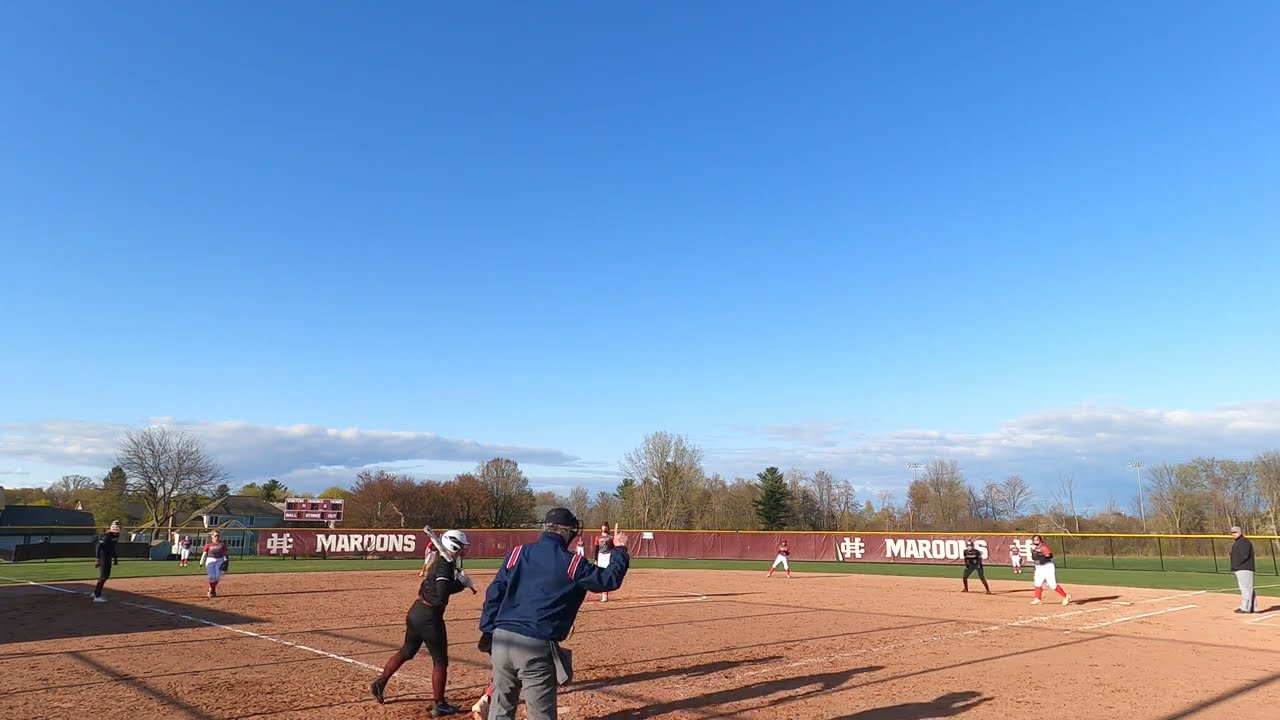The image depicts a high school baseball game in progress, taken from the perspective of the pitcher. The field is characterized by its light brown sandy dirt with white lines outlining the bases, home plate, and pitcher's mound. Surrounding the field is neatly trimmed green grass and a black chain-link fence topped with yellow padding. Maroon-colored banners with "CH" and "Maroons" emblazoned on them are affixed to the fence.

In the foreground, an umpire dressed in a blue jacket, gray pants, and a black hat is seen with his right hand raised, index finger pointing up, possibly signaling a strike or giving instructions. A batter, dressed in an all-black uniform and equipped with a helmet, stands ready at the plate. The opposing team is attired in black and red jerseys with white pants.

The surrounding area features several rectangular houses with gray roofs visible in the distance, adding to the charming small-town atmosphere. Above, the sky is a light blue, dotted with visible white clouds. On the other side of the fence, a few trees, still bare as if early in spring, add a touch of nature to the scene. The game appears to have just started, with the teams poised for the next play.